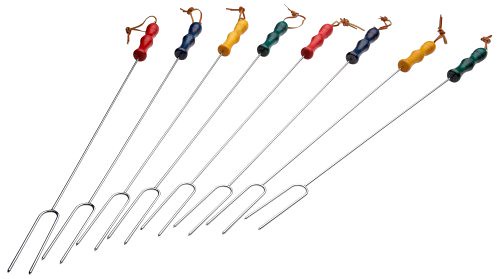This photograph displays an assortment of eight long, metal, two-pronged forks designed for roasting hot dogs over a fire or grill. The white background highlights the vibrant colors of the rounded, lathed wooden handles, which come in pairs of red, blue, yellow, and dark green. Each handle features ergonomic grooves for easy grip and a knotted leather loop at the end, which can be useful for hanging or securing the utensils. The main part of these forks is constructed from straight silver metal, which extends into a distinctive elongated arch ending in two small-pronged tips, suitable for skewer-like tasks and ensuring hot dogs are securely held. These versatile prongs facilitate even cooking and manipulation of food over an open flame, making them ideal for both kebab house skewer uses and campfire cooking.